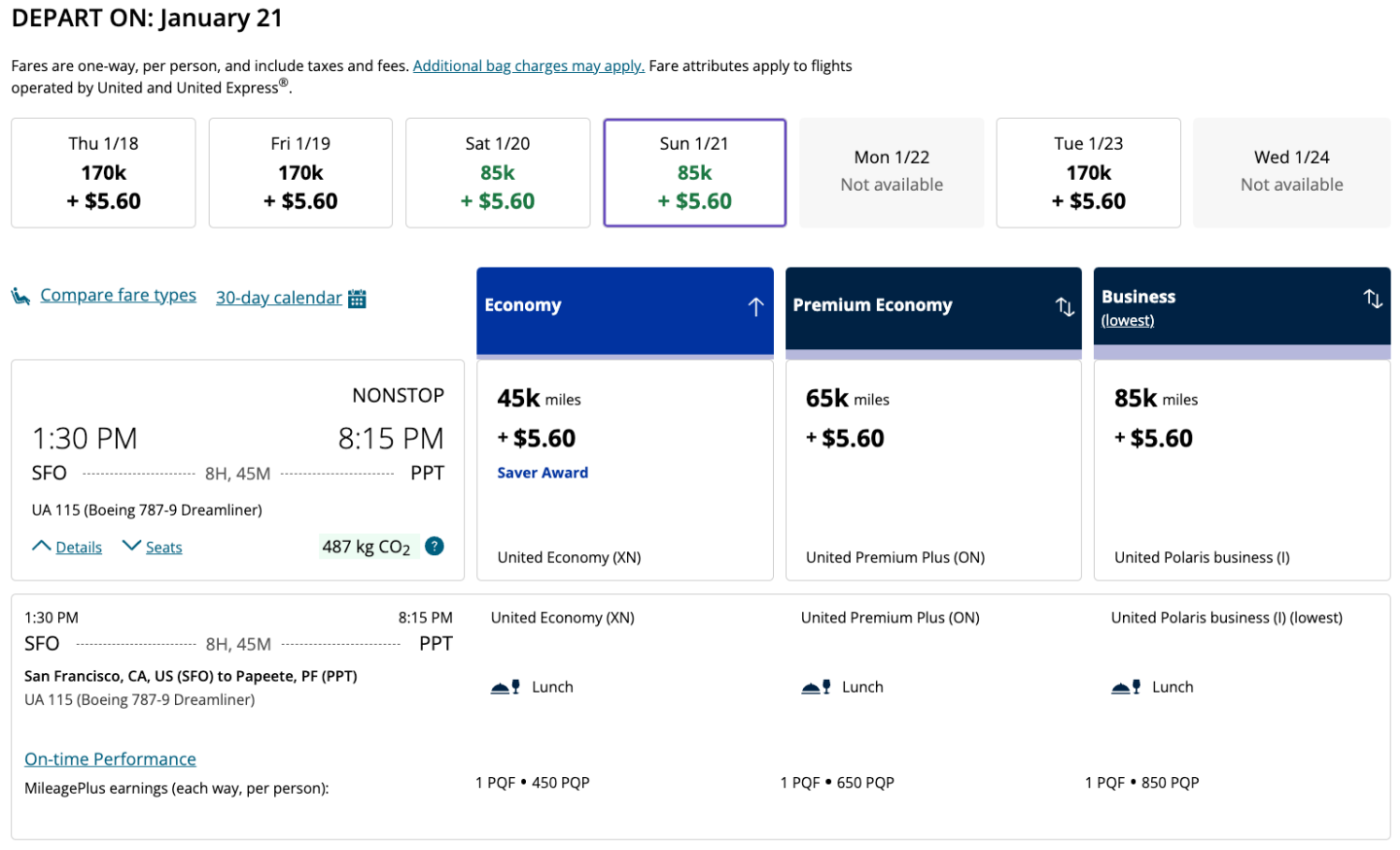The image appears to be a screenshot of an airline booking service, specifically the section where users can select their flight dates and view pricing details. At the top left corner, there is an option to "Depart on January 21st." The date range displayed spans from Thursday, January 18th to Wednesday, January 24th. 

For each date, the costs are as follows:
- Thursday, January 18th: 170k miles plus $5.60 
- Friday, January 19th: 170k miles plus $5.60
- Saturday, January 20th: 85k miles plus $5.60
- Sunday, January 21st: 85k miles plus $5.60
- Monday, January 22nd: Not Available
- Tuesday, January 23rd: 170k miles plus $5.60
- Wednesday, January 24th: Not Available

Below this date range, specific flight details are provided:
- Departure Time: 1:30 p.m. from SFO (San Francisco International Airport)
- Duration: 8 hours and 45 minutes
- Flight Type: Non-stop
- Arrival Time: 8:15 p.m. at PPT (Fa'a'ā International Airport, Tahiti)

These details are arranged in a clear, structured manner to help the user compare flights and make an informed decision.